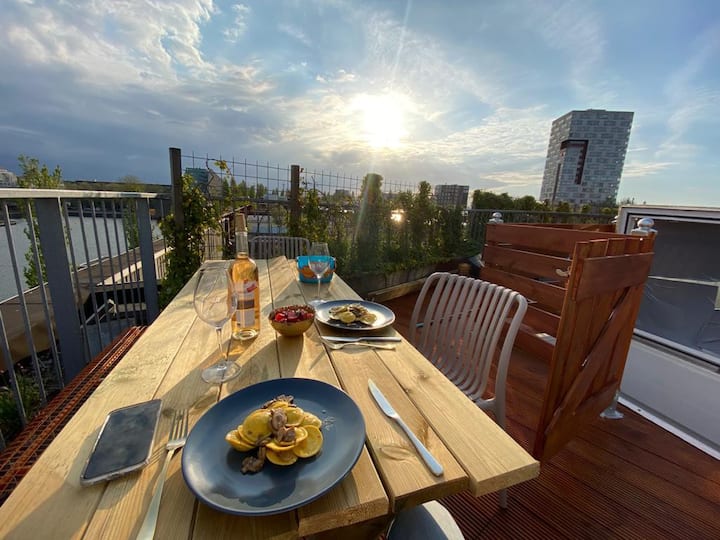This vibrant outdoor colour photograph captures a charming rooftop dining scene, set against a semi-cloudy, light blue morning sky with the hazy sun peeking through the clouds. Centered in the composition is a rustic wooden table made up of planks, situated on wood-paneled flooring. A metal chair with numerous railings is tucked neatly on the right side of the table, creating an inviting atmosphere. Spread across the table are dark blue plates and bowls, each brimming with beige and brown-colored food that resembles ravioli with sauce. Complementing the setting are a wine glass and a bottle of rosé wine at the table's center, along with another empty wine glass placed by each plate. 

A small red bowl, possibly containing fruit, is positioned in the middle, flanked by light-green stems, and there is a blue bucket with a handle at the far end of the table. Personal items include a phone placed towards the left corner. The background reveals lush foliage and the silhouette of a large building in the upper right-hand corner, framed by a metal fence and a wooden gated structure, enhancing the rooftop's cozy and secluded ambiance.